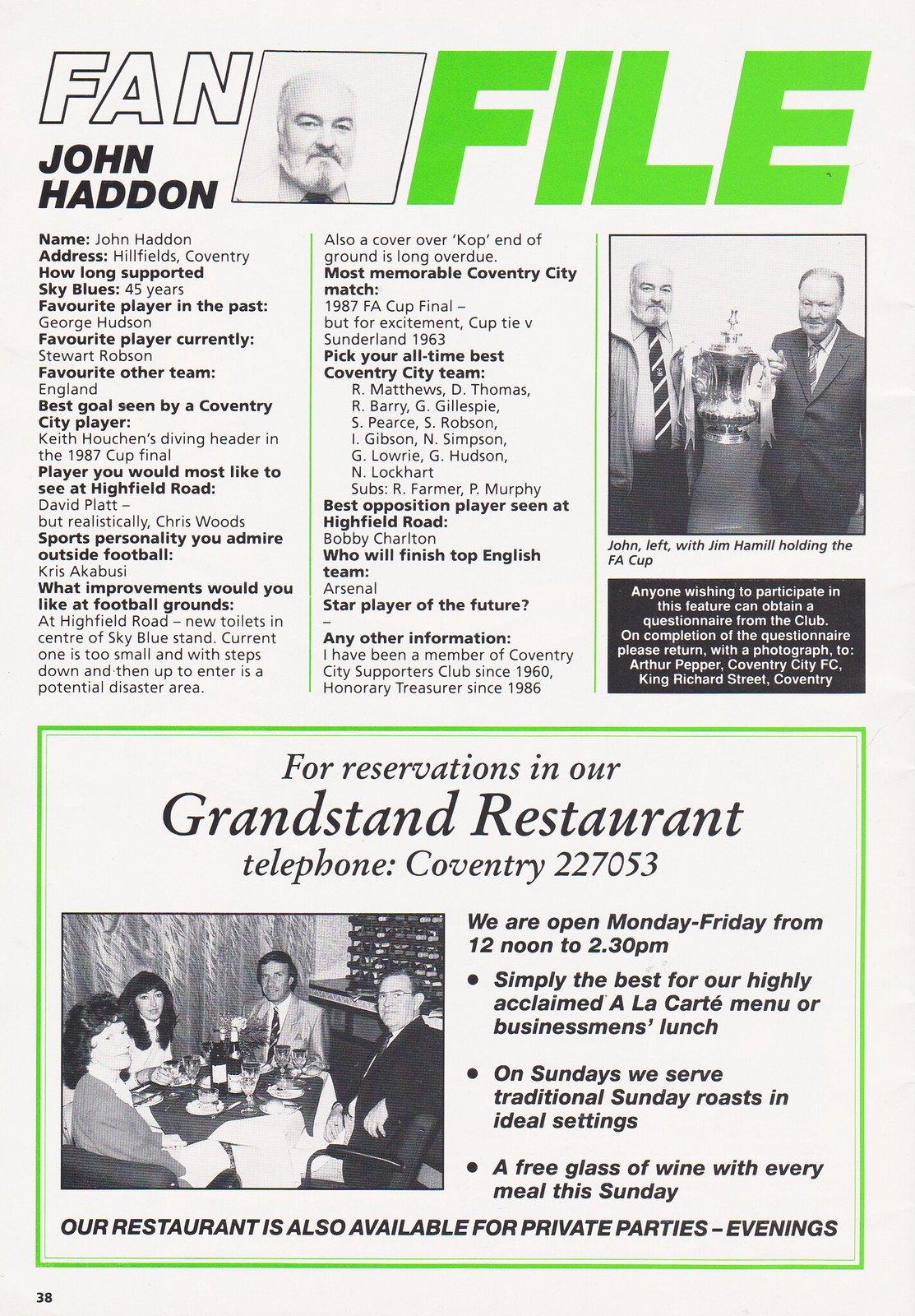This vertically oriented image resembles a newspaper feature titled "Fan File," prominently highlighted in large green block letters at the top right. In the upper section, a black-and-white photograph of a partially bald man with a white mustache and beard is situated next to the title, emphasizing the fan, John Haddon. To the left of this image, in bold black letters, is “John Haddon.” Below his name, a detailed profile includes his personal information and preferences such as name, address (Hillfields, Coventry), and extensive details about his support for the Sky Blues for 45 years.

The profile elaborates on John Haddon's favorite past player (George Hudson), favorite current player (Stuart Robson), and other favored teams (England). It mentions his best goal seen, Heath Hootchins' diving header in the 1987 Cup Final, and his desired players for Highfield Road: ideally David Platt, and more realistically, Chris Woods. Additionally, it lists sports personality Chris Akabusi as someone he admires outside of football, and discusses improvements he wishes to see at the football grounds, particularly new toilets in the center of the Sky Blues stand due to the current ones being inadequately small and hazardously designed.

A thin vertical green line sections off the right side of the page where a larger square photograph appears below the word "File.” This image shows John Haddon in a suit and tie, holding one side of a trophy alongside another formally dressed man.

At the bottom, a large rectangular advertisement with a green border invites readers to make reservations at the Grandstand Restaurant by calling Coventry 227053. This section details their opening hours (Monday to Friday from noon to 2:30 p.m.) and highlights their offerings, including a highly acclaimed a la carte menu and traditional Sunday roasts, with a promotional note on a complimentary glass of wine with every meal this Sunday. The advertisement features a black-and-white photo of two couples dining in the elegant setting of the restaurant.